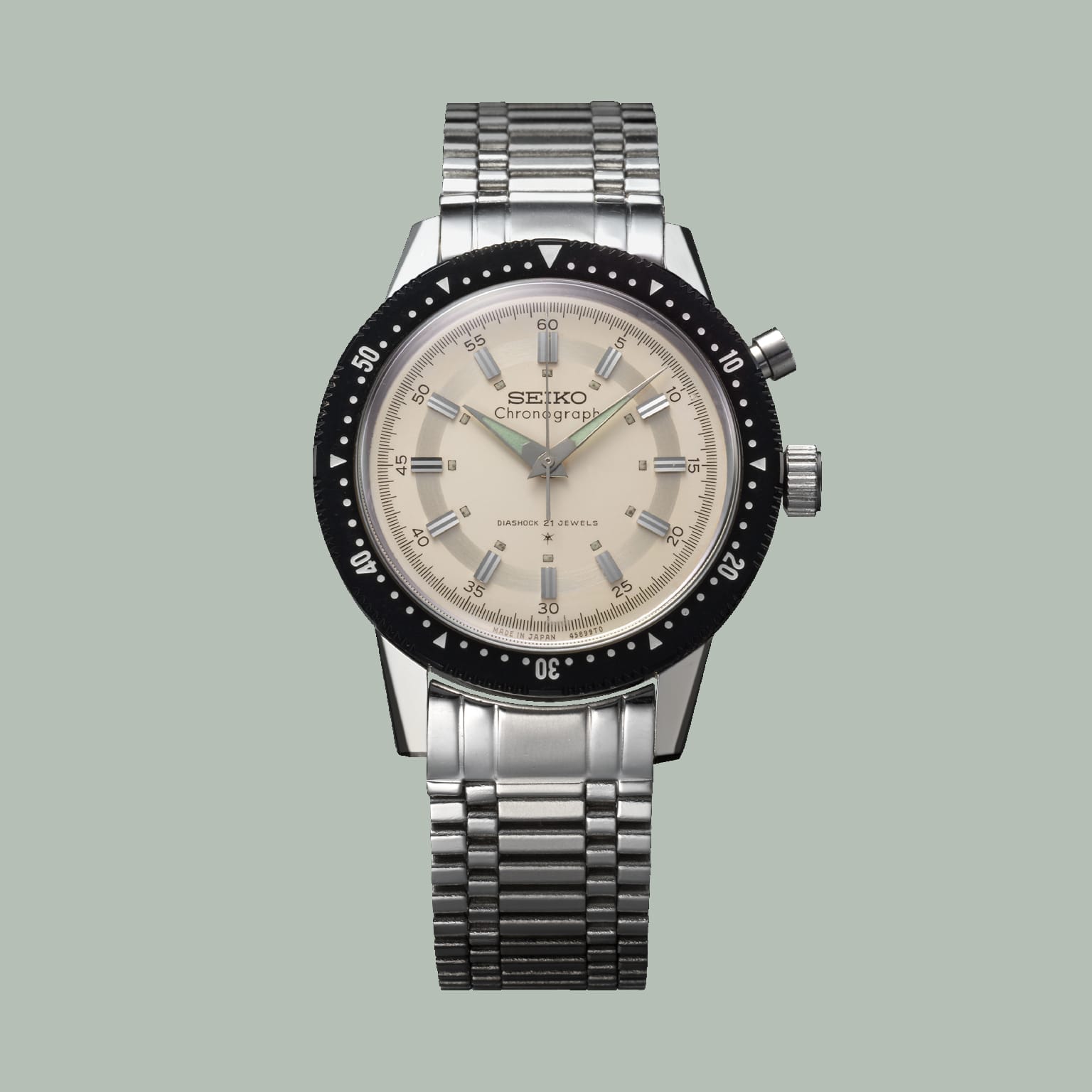This image showcases a Seiko chronograph men's watch with a distinctive silver metal link band, set against a grayish-green, square background. The watch features a large, off-white face adorned with intricate details and Roman numerals. Surrounding the watch face is a black dial marked with increments of 10, 20, 30, 40, and 50, and interspersed with smaller white dots. At the top of the dial, there's a prominent triangle indicating the 60-minute position. The watch hands, which might be glow-in-the-dark, are uniquely arrow-shaped, adding a precise touch to the design, with the time set at 10:08. Two knobs are positioned on the right side of the watch face for additional functionality. The watch's face is reflective due to a light shining on it, emphasizing its elegant and coordinated design.